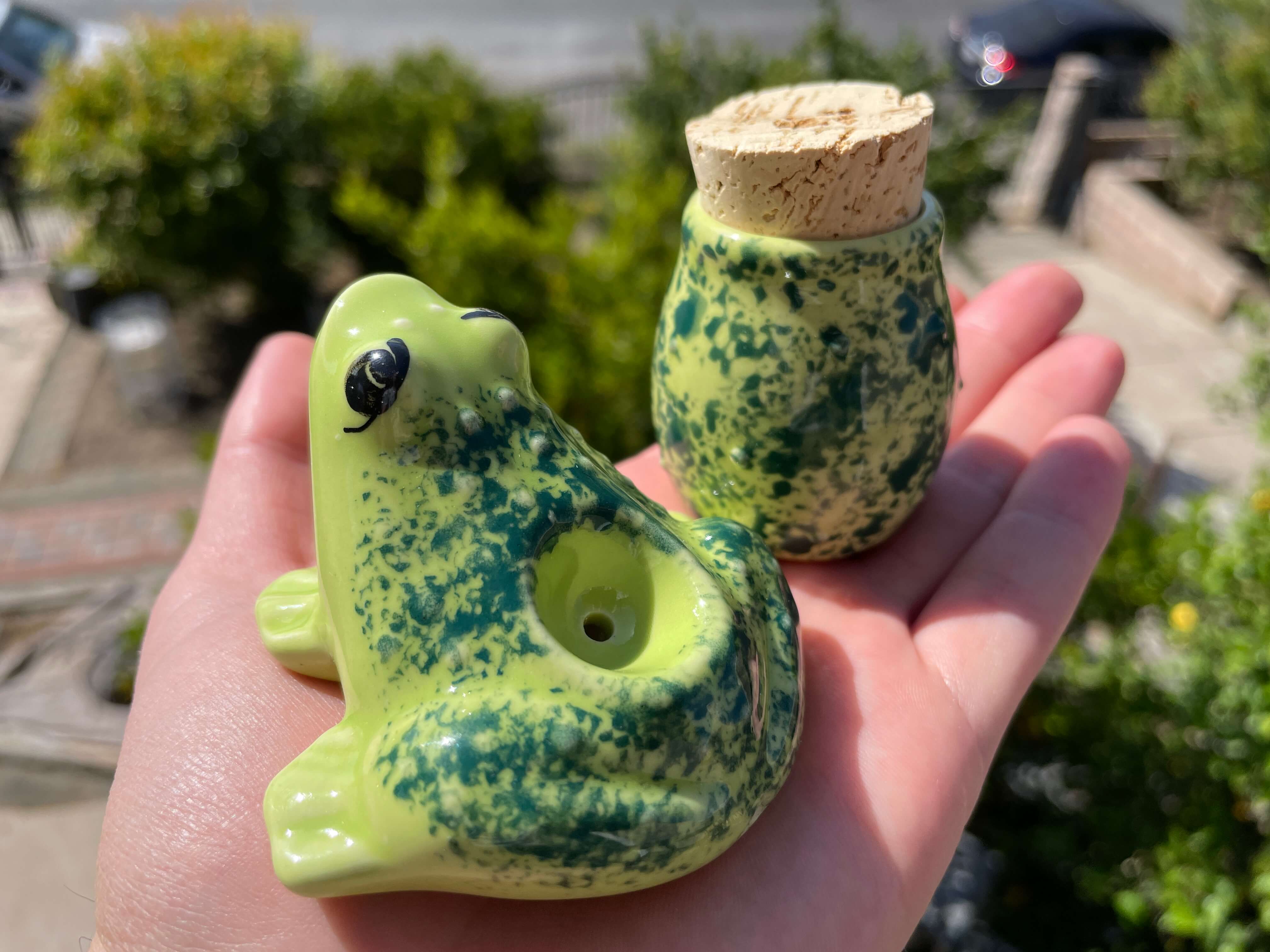The image prominently features a left human hand extended flat and holding two distinct, similarly colored objects. The focus is on a light yellow, ceramic frog with dark green speckles scattered across its body. The frog is positioned near the front of the image, with a concave circular indentation at the top, which is likely intended for use as a smoking pipe. Its face is oriented upwards, and on the left side, it has a black eye. Adjacent to the frog, on the right side of the hand, rests a small, round ceramic container that mirrors the frog's lime green color and dark green speckles. This container is capped with a cork lid. The background appears to feature a garden pathway leading down to a street, adding a natural setting to the scene.